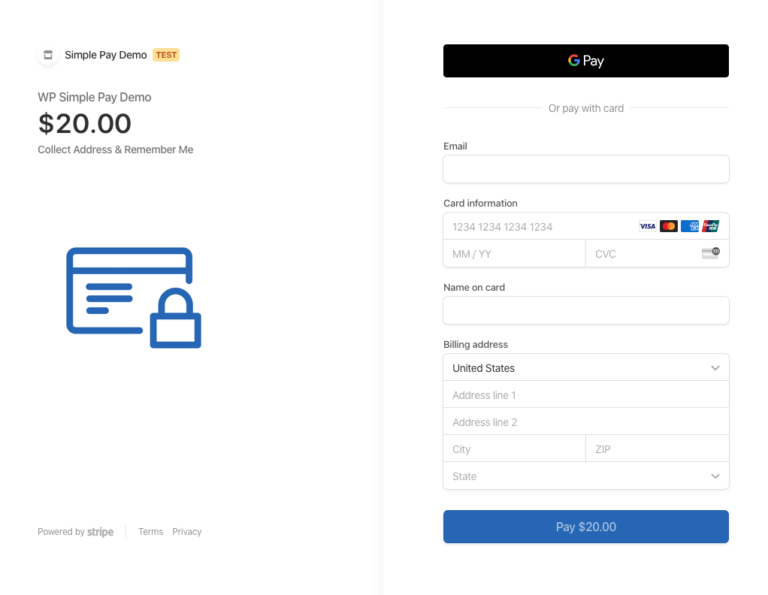The image consists of two evenly divided mobile screenshots with a thin gray border separating them vertically. 

On the left screenshot:
- The background is entirely white.
- In the top-left corner, there is a white circle with a gray calendar icon inside it.
- To the right of the calendar icon, "Simple Pay Demo" is written in black text.
- Below this, an orange tab with dark orange text displaying the word "Test" is visible.
- To the left and slightly downward, "WP Simple Pay Demo" is noted in black text in large fonts.
- Below this, "$20" is inscribed in big, bold letters.
- Underneath this, the text reverts to regular print displaying "Collect Address" and "Remember Me."
- A blue address icon is present with a blue lock icon situated in the bottom-right corner.
- In the lower-left corner, in small black print, it reads "Powered by Stripe."
- In the center-bottom of the screenshot, "Terms" and "Policy" are listed with a space between them.

On the right screenshot:
- This screenshot also features an entirely white background.
- At the top, there's a black tab that includes a Google "G" icon and "Pay" written in white text next to it.
- Below this, it states "Or pay with card" in black text.
- Next, there's a field for inputting an email address, denoted by a long rectangle.
- Following the email field is a section for card information, including a long rectangle for the card number.
- Beneath this are two smaller fields side-by-side for the month and year on the left, and the CVC on the right.
- Further down, it says "Name on Card" in black text with a designated rectangle for the input.
- Next is the billing address section, featuring multiple rectangles for inputting the address.
- Finally, at the bottom, there's a blue button with "Pay $20" centered inside it.

This meticulously detailed caption provides a comprehensive description of the given mobile screenshots.